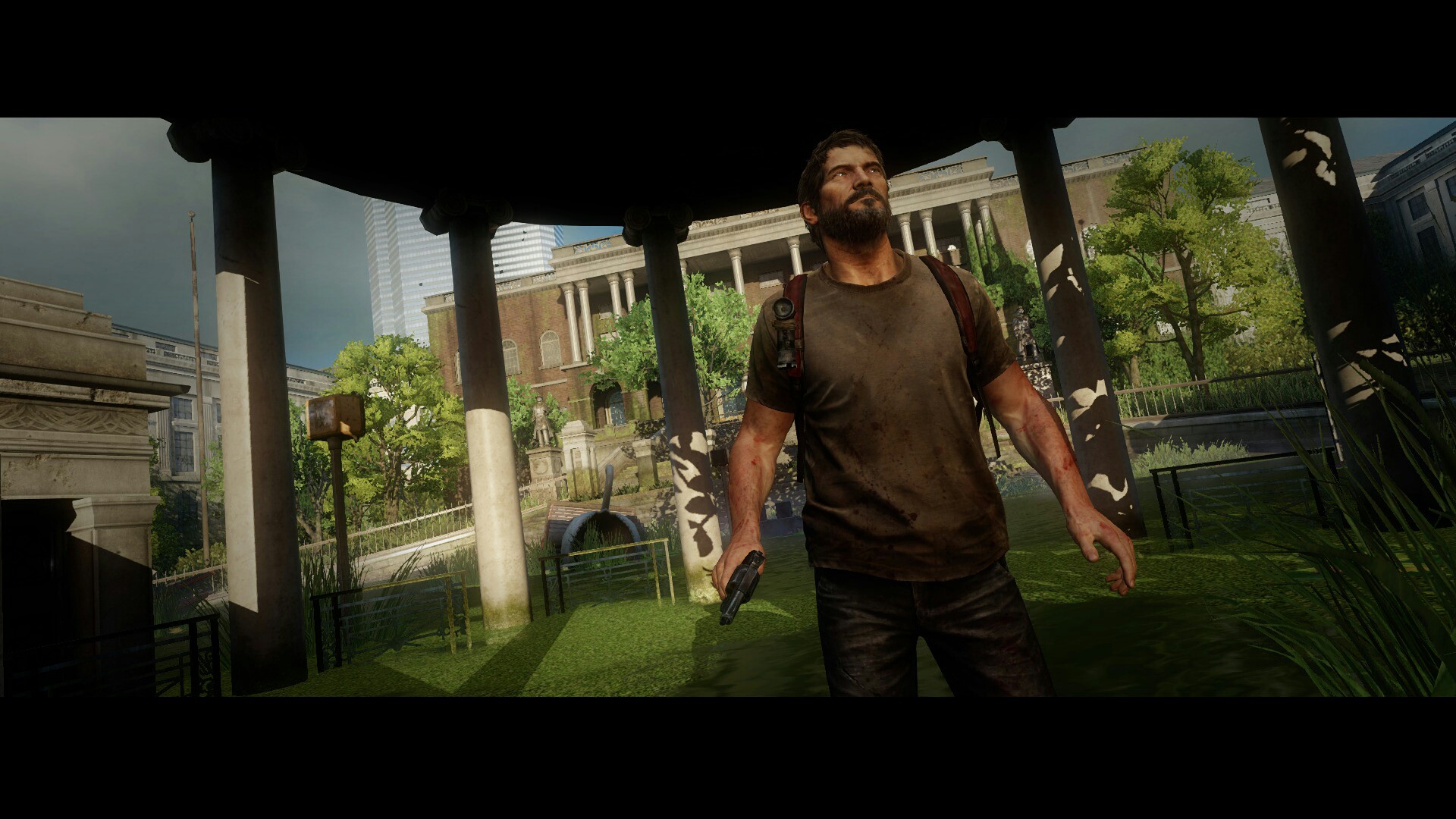The image showcases a high-quality screenshot from a video game. In the foreground, a rugged, animated male character stands on a grassy area, equipped for a potential confrontation. He wears a distressed brown t-shirt, dark pants, and carries a brown backpack over his shoulders. In his left hand, he grips a pistol, his right hand positioned slightly forward, revealing a mustache, beard, and short brown hair as he looks upward.

The setting features the character under a gazebo with white pillars, situated centrally in the image. Surrounding the gazebo are tall buildings; one dominant structure in the background and another visible on each side. The scene also includes some scattered weeds on the grass. The top and bottom of the image have black borders, reinforcing the focus on the central action. The background combines digitally rendered elements with realistic touches, such as a bluish-gray sky peeking through and some visible trees, enhancing the immersive environment.